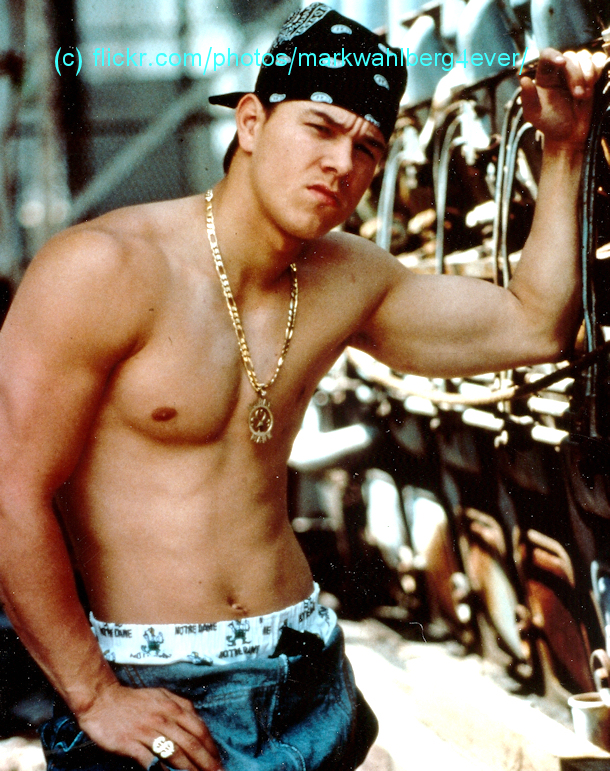The image features a shirtless, muscular Caucasian man with a confident, almost cocky scowl reminiscent of a young Leonardo DiCaprio or Mark Wahlberg. He is wearing dark blue jeans with the waistband of his white boxers slightly revealed, displaying a dark-font "Notre Dame" and a lion design. Around his neck, he sports a thick gold chain with a round pendant. His left arm, adorned with a dollar-sign ring, rests on one of his legs, while his right forearm leans against a wall, indicating a self-assured posture. He completes the look with a bandana tied around his head. The top of the image displays blue text that reads: “(C) flickr.com/photos/MarkWahlbergForever/.”